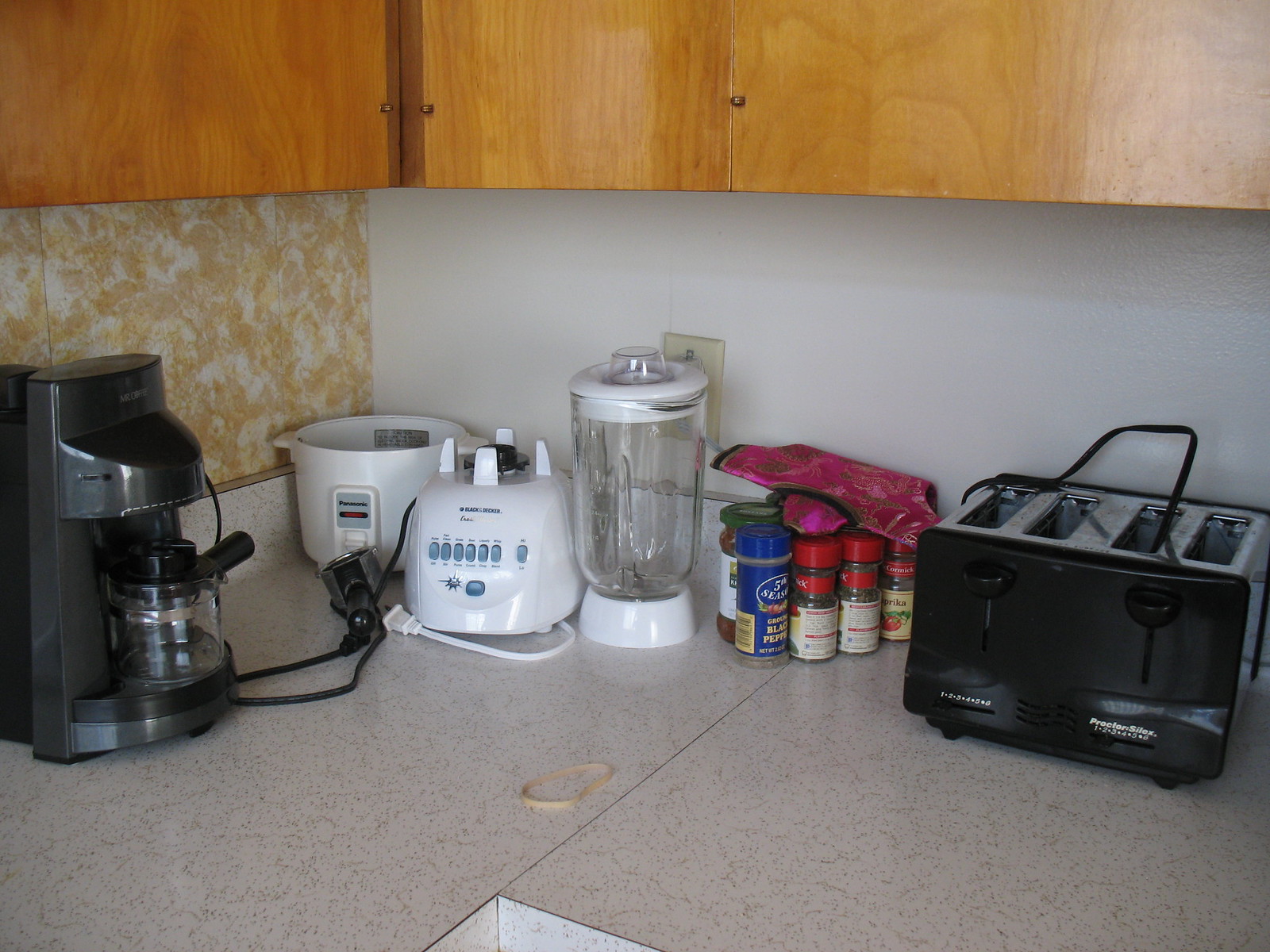The image captures a corner section of a kitchen countertop made from white granite. The countertop extends in two directions: to the right and left, creating an L-shaped corner. On the left side of the countertop, the wall features a wallpaper with a predominantly white background accentuated by irregular gold blotches. In contrast, the wall on the right side is covered with a plain white wallpaper.

Above the countertops on both sides are brown wooden cabinets, creating symmetry in the kitchen's design. On the left, the cabinet is mounted above the white and gold patterned wallpaper, while on the right, another brown wooden cabinet is positioned above the plain white wall.

The countertop itself is populated with various kitchen appliances and items. A toaster, several seasoning containers, and a blender with its base separated are placed on the counter. Additionally, a coffee pot rests on its base, ready for use.